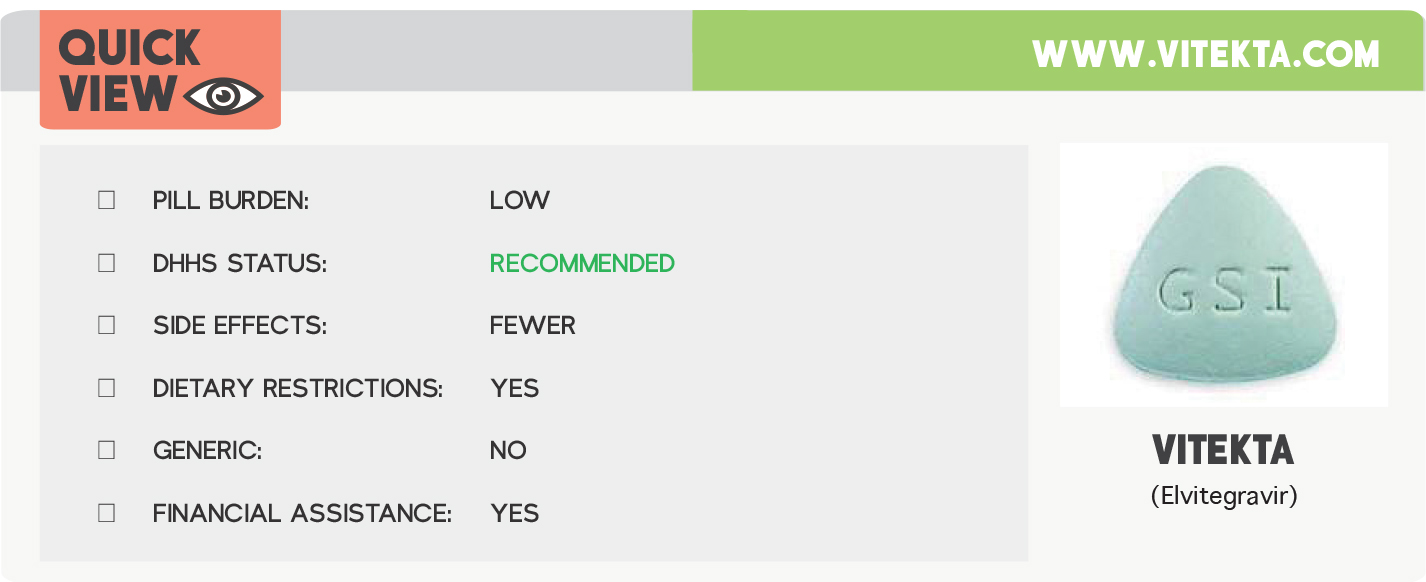This screenshot displays the user interface of the website www.vitekta.com, which is spelled "V-I-T-E-K-T-A". The website name is prominently presented in white text against a green banner at the top of the image.

To the left of the main content, there is a gray sidebar featuring a "Quick View" button. This button includes a small, dark peach-colored eyeball icon.

Dominating the main section of the screenshot is a large gray box, which is divided into six options. Each option includes a small square checkbox for potential selection. These options are detailed as follows:

1. **Pill Burden**: Low
2. **DHH Status**: Recommended (the term "Recommended" is highlighted in green)
3. **Side Effects**: Fewer
4. **Dietary Restrictions**: Yes
5. **Generic**: No
6. **Financial Assistance**: Yes

Adjacent to this list, on the right side of the gray box, is an image of the pill. The pill is green and triangular, with "GSI" imprinted on its front surface. Below this image, the text "VITEKTA" is displayed, followed by "Alida Grevier" in parentheses.

This detailed presentation provides a clear view of the website's layout and key features related to the medication VITEKTA.